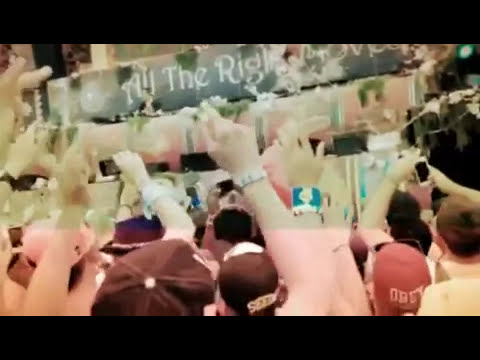The image appears to capture a blurred, somewhat distorted scene of a crowd gathered outdoors. The colors of the photograph are faded, giving it an older, almost sepia-toned feel. The people, with their backs to the camera, have their arms raised in the air, appearing to cheer or celebrate, with several capturing the moment on their smartphones. Among the crowd, many are wearing baseball caps in maroon and red colors. In the background, thin, rectangular objects resembling large book spines dominate the scene. The topmost object is painted black with white lettering that reads "all the right," albeit torn, while the one below is light red with black and white stripes, followed by a few more similarly colored objects. The entire image has an unnatural color effect, with a pink hue at the bottom transitioning to a tan shade at the top. Additionally, there are black rectangular strips bordering the top and bottom.